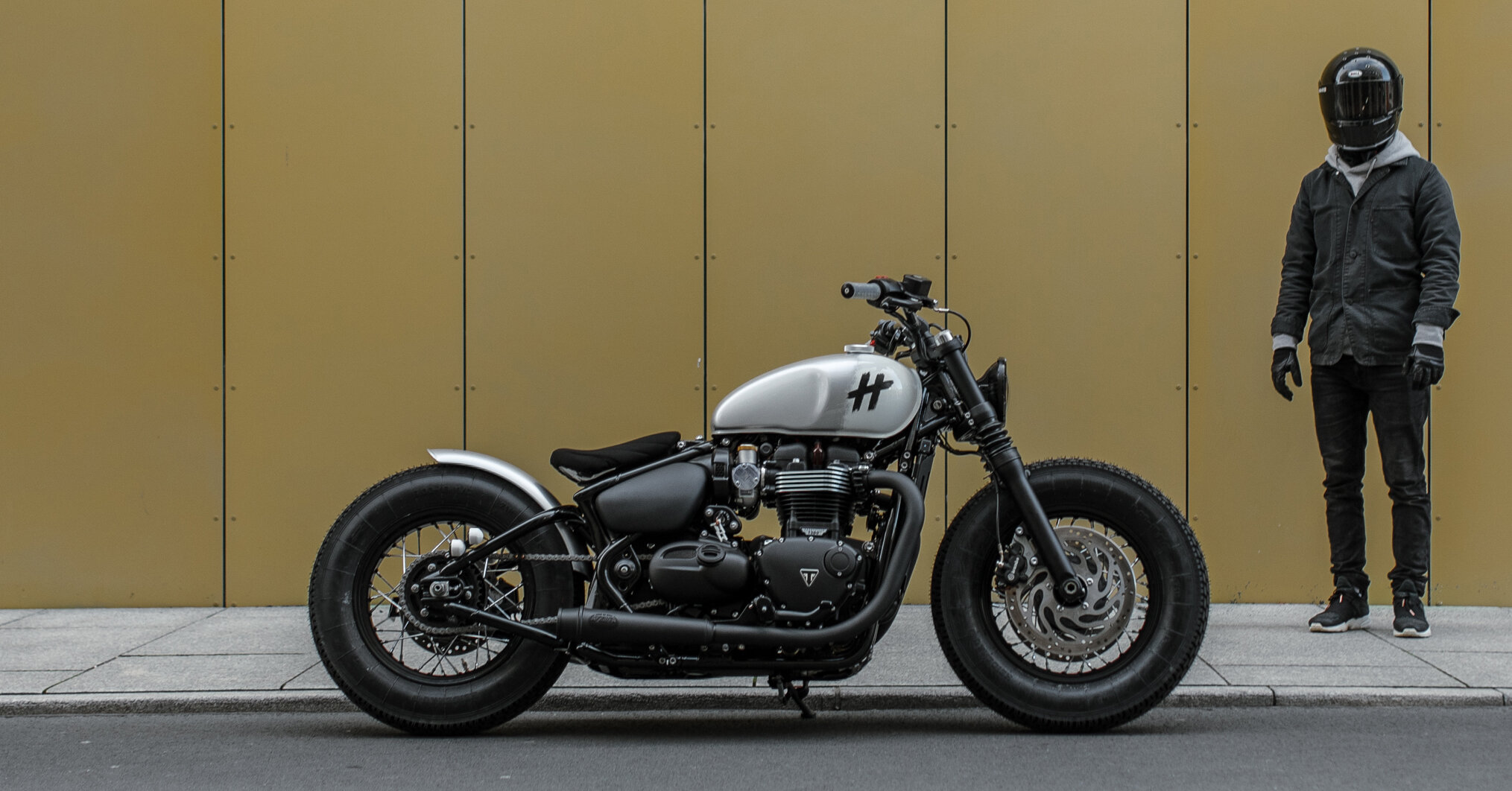The photograph captures a detailed scene featuring a motorcycle parked on a light black asphalt street near a light gray sidewalk. Central to the image is a Triumph Bonneville Bobber motorcycle, which showcases a striking combination of black and silver, including its silver gas tank and black tires. The motorcycle's silver handlebars and full view of the front and back wheels are clearly visible.

To the right side of the image, a man stands on the sidewalk wearing a distinctive charcoal gray jacket over a light gray hoodie, black skinny jeans, black gloves, and black tennis shoes with white soles. His face is obscured by a black helmet with a black visor. The backdrop reveals a wall adorned with six gold panels, adding an interesting contrast to the overall scene.